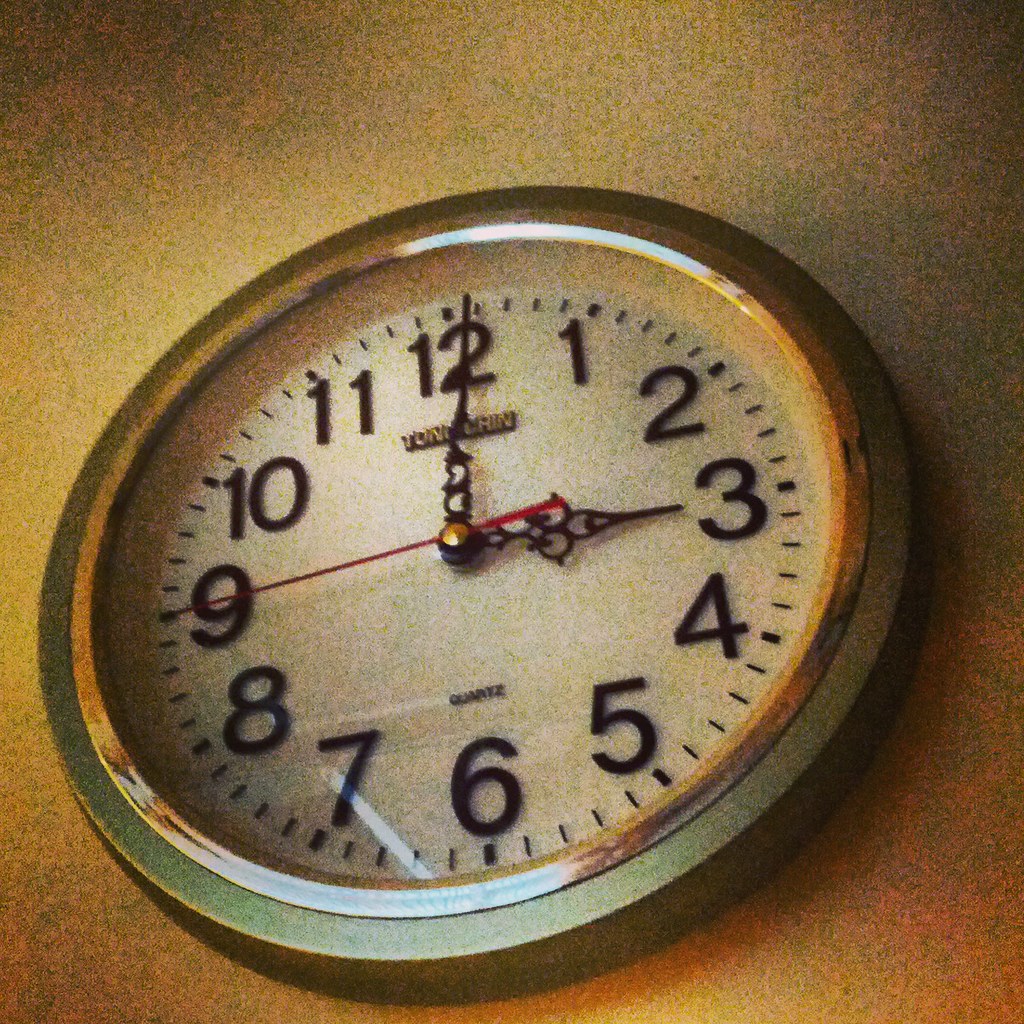This image depicts an old-fashioned, round analog clock mounted on a somewhat grainy, dimly lit yellowish wall. The clock features a greenish-gray frame with a slightly metallic inner rim, appearing silver or gold, likely due to reflections. The clock face is white with bold black numbering from 1 to 12. The hour and minute hands are intricately designed with black, lace-like iron work, while the long slender second hand is red, extending to the 9. At the time of the photo, the hour hand points to 3, the minute hand is just past 12, and the second hand is almost touching the 9, indicating approximately 3:01 and 45 seconds. There is a partially obscured logo near the 12 that might read "Jan Rin" or similar, and the word "Quartz" is visible above the 6.